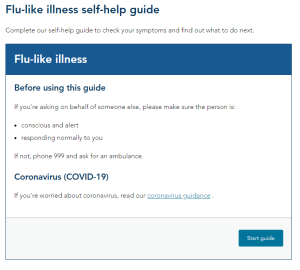This smaller, square-shaped image appears to be a screenshot taken from a health website, featuring a clean, white background. Positioned on the left side is a prominently displayed title in dark blue font that reads "Flu-Like Illness Self-Help Guide." Just below the title, a brief description is provided in gray text, which says, "Complete our self-help guide to check your symptoms and find out what to do next."

Beneath this description, there's a distinct, square-shaped text section outlined in a dark blue color with a thicker header also in dark blue. The header bears white text stating "Flu-Like Illness." Below this header, the section contains a rectangular area with a white background and additional details. In blue text, it reads, "Before using this guide," followed by gray text informing users, "If you're asking on behalf of someone else, please make sure this person is:" There are two bullet points listed in gray text: "Conscious and alert" and "Responding normally to you." Further instructions state, "If not, phone 999 and ask for an ambulance."

The guide also includes a section titled "Coronavirus (COVID-19)" in dark blue text, followed by gray text advising, "If you're worried about coronavirus, read," with an underlined, blue clickable link that says "coronavirus guidance."

Finally, on the lower right portion of the image, there is a rectangular, blue button with white text that reads "Start Guide."